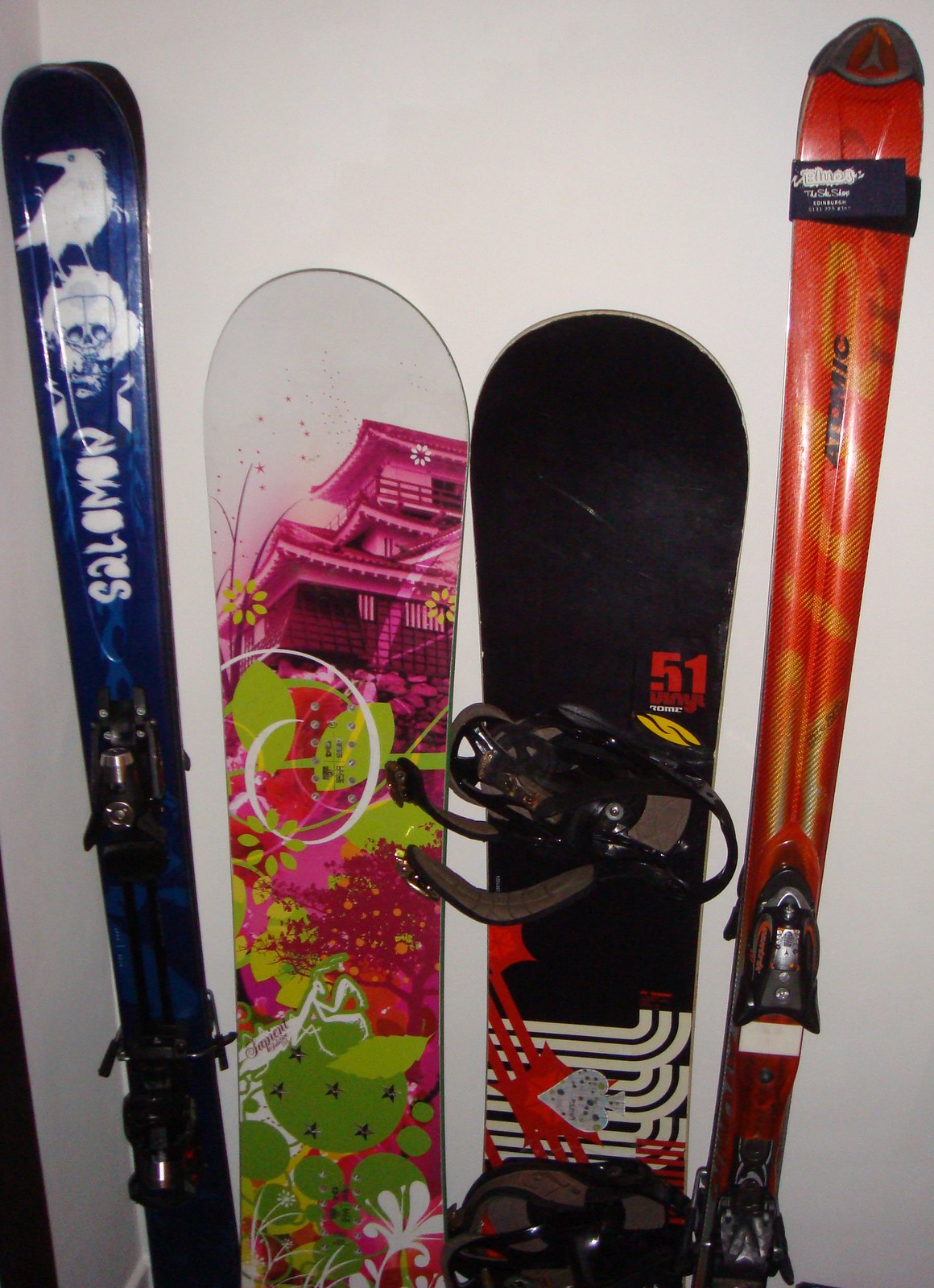The photograph captures a collection of skiing and snowboarding equipment arranged against a white wall. From left to right, the lineup includes a blue Salomon ski featuring a white graphic of a bird perched on a skull, a snowboard showcasing a Japanese house design in pink with flowers and plants beneath it, a black snowboard adorned with white line logos and a red '51', and a red Atomic ski which lacks any distinct graphics. The equipment appears well-worn, with bindings on the skis set at different positions, indicating varied lengths. The first snowboard's binding is either turned away or missing, while the second snowboard has its binding visible. The two skis are secured together with straps at the top, highlighting their functional lengths and usage. Despite the poor lighting, the vivid details and intricate designs on the skis and snowboards create a visually engaging scene.